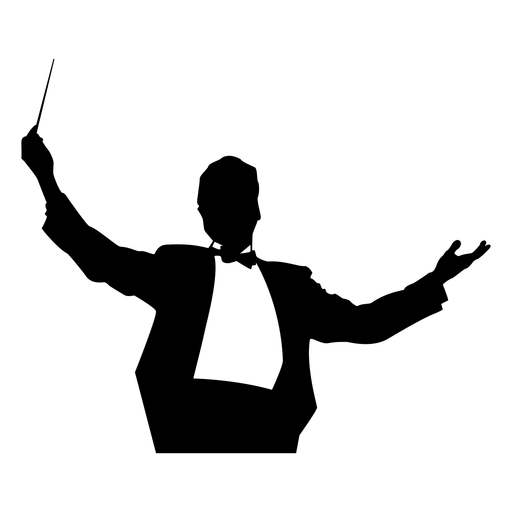This black-and-white illustration shows the silhouette of a man, likely a composer or conductor, depicted from his upper thighs to his head. He is dressed in a tuxedo, with a white shirt and a black bowtie, and his face is entirely blacked out, with no discernible facial features. The conductor’s arms are raised in the air, with his left hand empty and his right hand gripping a baton, poised as if leading an orchestra. His body and clothing are primarily rendered in black, standing out starkly against the white background, emphasizing the simplified and abstract nature of the image. The silhouette lacks detail but clearly conveys the poised and dynamic energy of conducting.